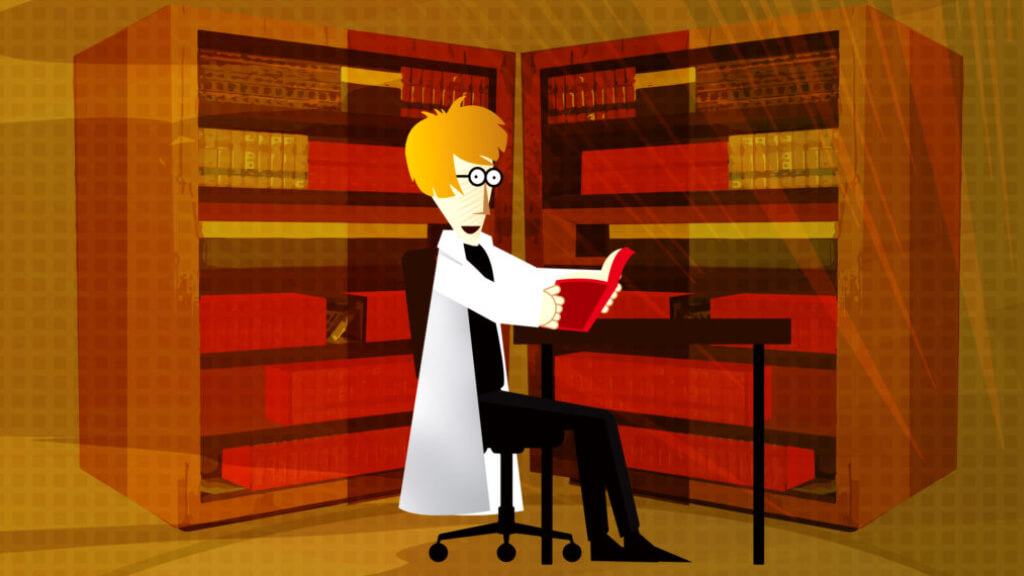This rectangular, approximately six-inch wide by three-inch high illustration features a cartoon scientist seated on a black, wheeled stool. The character is positioned centrally, with a thin desk or table in front of him. The scientist has an inverted triangular head with golden brown hair and black circular glasses, each lens featuring two dots for eyes. His face is characterized by a large, sharp, triangular nose and an open mouth that seamlessly blends with his neck, creating a tapering effect.

He is dressed in a long white lab coat, underneath which he wears black pants and a shirt. His arms are extended forward as he intently holds and reads a red book. The backdrop includes two large, minimalistic bookshelves—one to the left and one to the right—packed with featureless square books colored primarily in reds, browns, and yellows. These shelves almost meet at the center of the background. The room's walls and flooring are depicted in a brownish tone, overlaid with numerous small, transparent gray squares, adding a textured, grid-like effect. Additionally, light gray transparent beams rise diagonally from the lower right-hand corner towards the upper left, enhancing the dynamic, layered look of the scene.